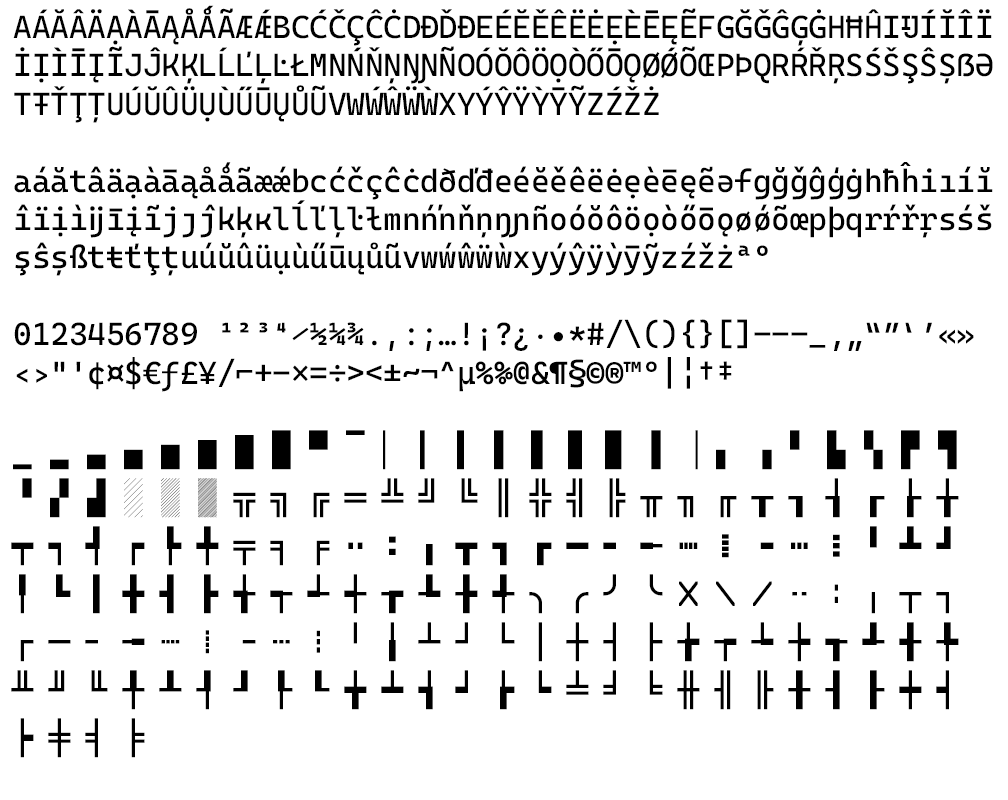The vertical image presents a detailed display characteristic of computer-generated text or coding symbols against a stark white background, likely the software interface's canvas. The content begins with an array of uppercase letters, each meticulously adorned with varying diacritical marks. For instance, the letter "A" appears in multiple forms: plain, accented, with an inverted breve, a circumflex, and an umlaut. This pattern of diverse symbols applied to alphabetic characters repeats across the entire uppercase alphabet, followed by a similar arrangement of lowercase letters.

Progressing further down the image, a sequence of numbers from 0 through 9 is displayed, consistent with their standard digital representation. This numerical array transitions into familiar symbols that populate a typical computer keyboard, including the hashtag (#), asterisk (*), question mark (?), among others. Below the alphanumeric and common symbols section, the image concludes with several rows of more abstract or special characters, commonly utilized in various programming languages and symbolic notation. The organized presentation juxtaposes the structural precision of computer code with the visual complexity of typographic variations.